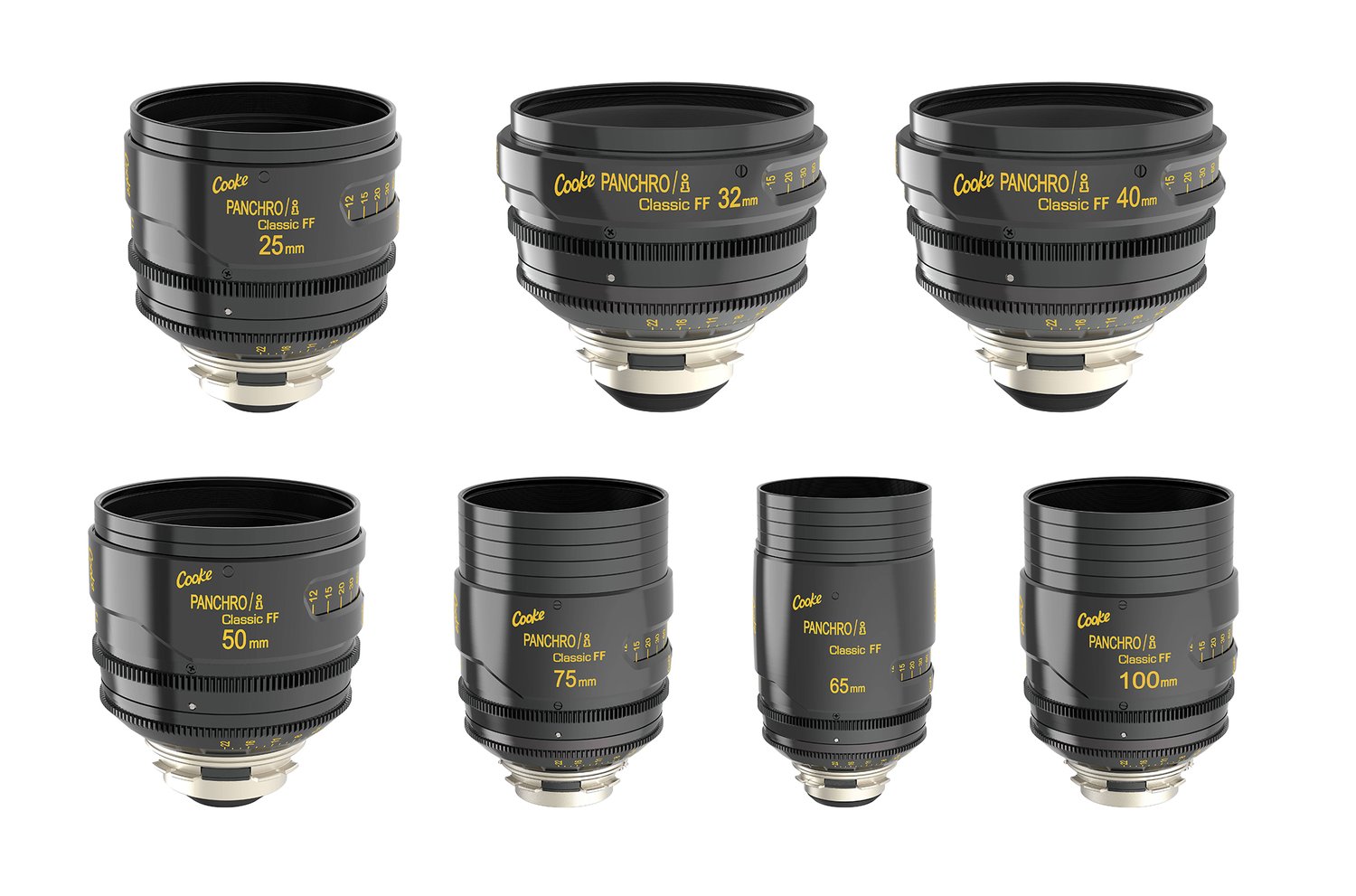This detailed photograph showcases an array of seven black camera lenses from the Cooke Company, each one neatly labeled with yellow text reading "Cooke Panchro Classic FF." The lenses are arranged in two rows: three wider lenses on the top row, measuring 25mm, 32mm, and 40mm from left to right, and four thinner lenses on the bottom row, measuring 50mm, 75mm, 65mm, and 100mm from left to right. Each lens has its respective millimeter size prominently displayed. Notably, the lenses in the bottom row have additional black rings on top of the initial lens structure. The bottom parts of these lenses feature a silver section followed by a black tip, giving a distinctive look reminiscent of the base of a light bulb.